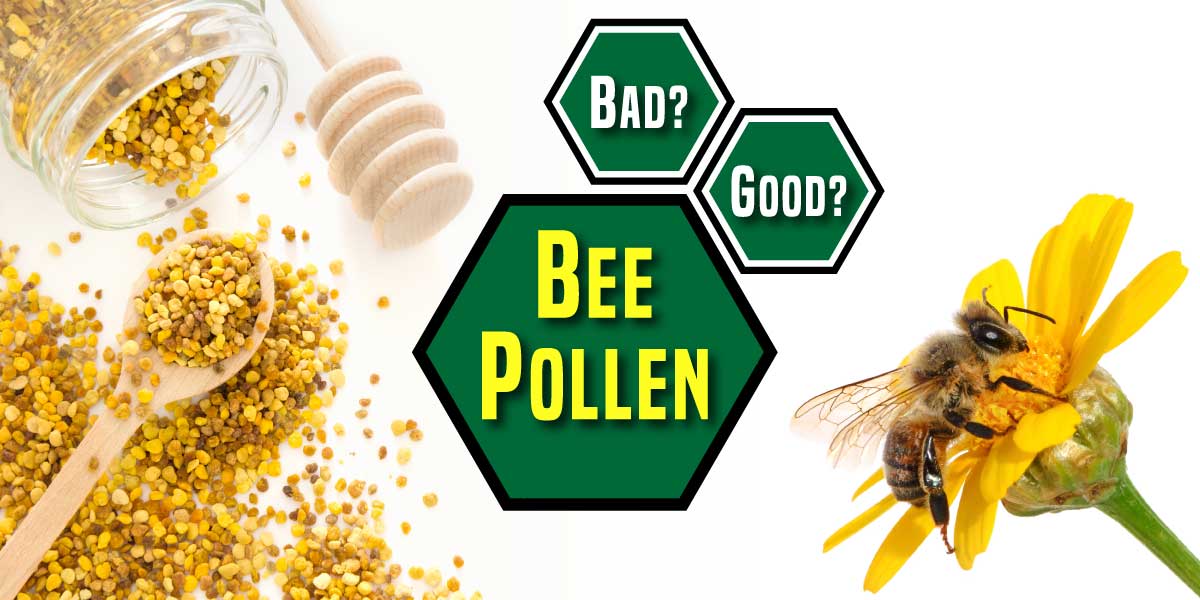The image is a detailed header for an article or advertisement about bee pollen, set against a clean white background. On the far left, there's a glass jar lying on its side, spilling out what appears to be granular bee pollen, characterized by its crunchy, pebble-like texture in various shades of yellow and tan. A wooden spoon, filled with these granules, extends from the lower left corner, hovering over the scattered pollen. Accompanying the jar is a traditional wooden honey dipper.

In the center of the image, three hexagon-shaped elements, reminiscent of bee hive cells, dominate the composition. The largest central hexagon, in green, features the words "bee pollen" in prominent yellow lettering. Flanking it are smaller hexagons with green backgrounds and white text, one asking "bad?" and the other "good?".

To the far right, there's a vivid image of a bee actively engaged in pollination on a bright yellow flower, anchoring the right side of the layout. The image combines these natural and textual elements to create a visually engaging discussion on the qualities of bee pollen.